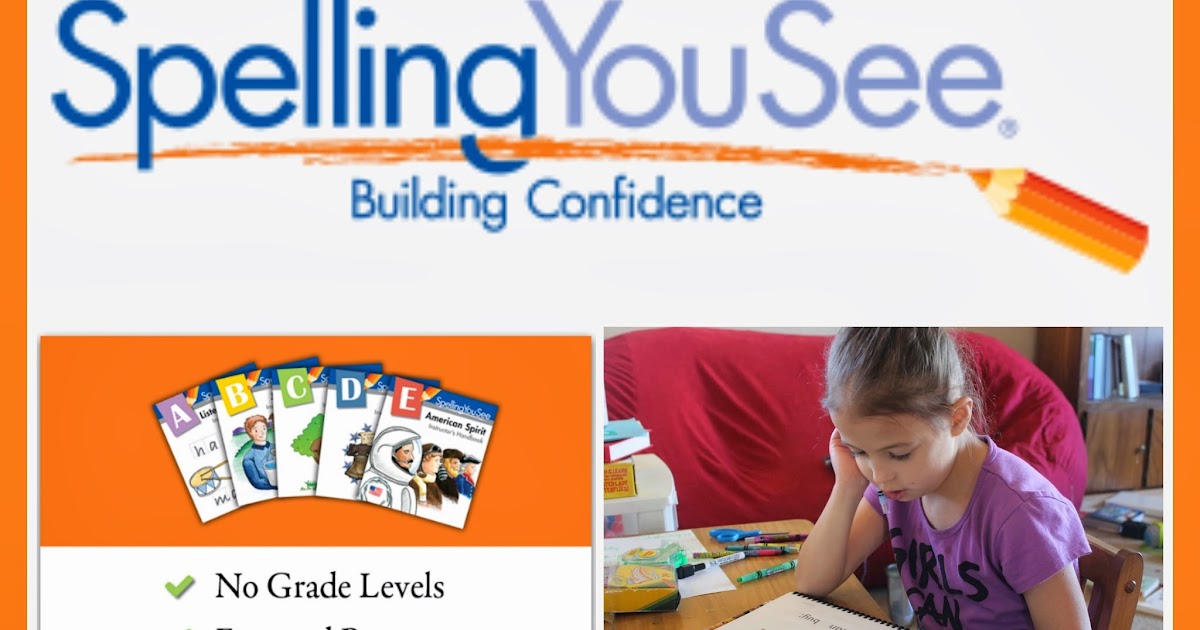This horizontal rectangular image features two thin vertical orange lines flanking either side. The primary background color of the image is white. At the top left, there is dark blue capitalized text that reads "SPELLING." To its right, there is slightly faded and blurry blue text that reads "UC," also capitalized. Below this text, an orange line spans the width of the image; it appears to be drawn with a colored pencil, specifically hinted by an orange colored pencil visible just underneath the "C."

In the center below the orange line, smaller blue capitalized text reads "BUILDING CONFIDENCE." At the bottom of the image, two different sections contain visual content. The bottom left section features an image with a black, orange, and white background, displaying various posters or magazines labeled from A to E. Underneath these labels is the black text "NO GRADE LEVELS," accompanied by a green checkmark to its left.

The bottom right section depicts a young white girl wearing a purple shirt with black text that says "GIRLS" and "OW" beneath it. She is leaning on a wooden desk, intently looking at something. The background includes a red couch, indicating it might be a living room setting. On the desk, identifiable items include green and red crayons, a pair of blue scissors, and some paper. Visible light reflections suggest the scene occurs during the daytime.